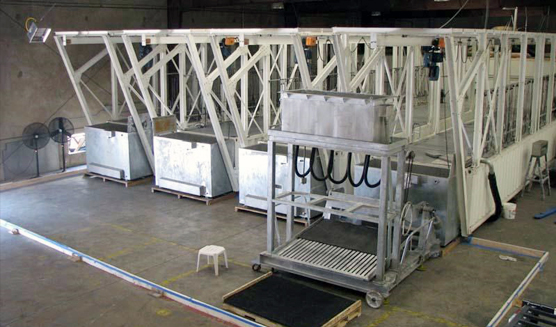In an indoor factory setting with concrete floors and walls, the image showcases four large, white, tunnel-like structures arranged close together. Each structure features a long rectangular metal bin with a significant opening at the end, resembling a conveyor system. These structures are supported by white steel bars, giving the appearance of uncovered bridges. Adjacent to the bins, there are larger-than-life metal rolling platforms that are reminiscent of grocery conveyor belts.

To the extreme right of the image, there's a distinctive metal apparatus with four black circular hoops extending downwards, accompanied underneath by what appears to be a plastic framework. This unit also includes additional metal bins situated on top. Encircling the entire assembly of white structures and the hoop apparatus, metal squaring creates a defined rectangular area on the factory's wooden floor.

Additional elements in the room include a small white plastic stool with four legs placed randomly to the left of the hoop apparatus. Also visible are two black standing fans positioned against the far left wall, and what seems to be a larger stool on the far right side. High above, there may be hanging equipment such as cameras. Furthermore, small orange lights can be seen on the upper parts of the white structures, adding to the detailed complexity of the scene.